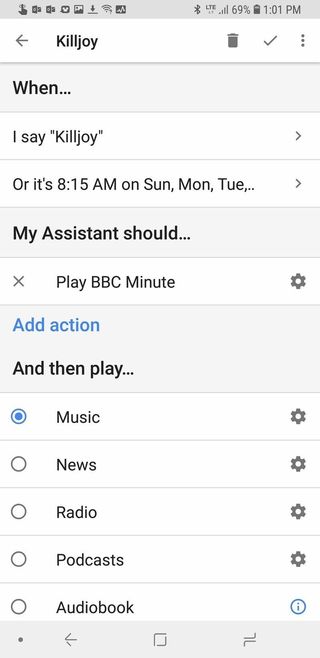The image displays a shortcut setup screen on a mobile device titled "Killjoy." At the top of the screen, there are navigational icons including a back arrow and a trash can icon to delete the shortcut, along with a checkmark indicating the shortcut’s confirmation. Directly below, the screen specifies conditions for when the shortcut should be activated: either when the user says "Killjoy" or at 8:15 PM on Sunday, Monday, and Tuesday. Further options suggest this schedule may extend to other days as well.

Following these conditions, the shortcut is configured to prompt the user's assistant to "Play BBC Minutes," with a settings icon adjacent to this action for customization. Below this, there's an "Add Action" button in blue which allows users to append additional tasks. The next section, labeled "And then play," offers various options such as music, news, radio, podcast, and audiobook. Each option is accompanied by a settings icon for adjustments, with the audiobook option featuring an additional information icon (an 'i' inside a circle) for more details. In the displayed configuration, the "Music" option is selected and highlighted in blue. The overall color scheme of the interface remains minimalistic, featuring primarily black and white, with blue accents on actionable items like the "Add Action" button, the information icon, and the selected "Music" option.